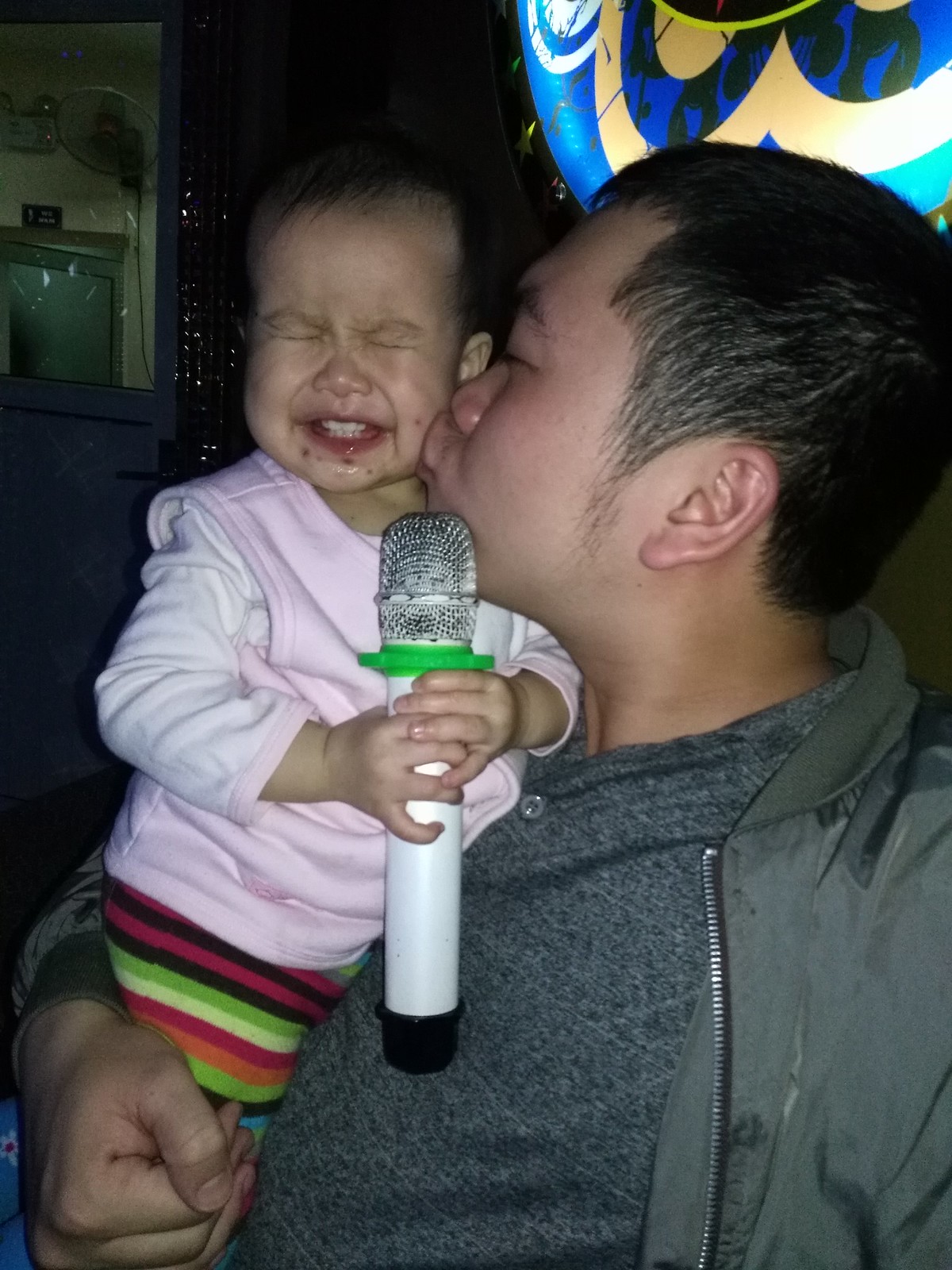In a heartwarming yet humorous moment, a man gently cradles a baby in his arms while planting a kiss on the baby's cheek. The baby, however, appears less than thrilled by the affectionate gesture. The man is dressed in a gray shirt paired with a gray jacket, exuding casual sophistication. The baby is adorably outfitted in a pink shirt and colorful shorts, gripping a distinctive white microphone adorned with a green band near the top and a black handle at the bottom. The background features a striking, brightly lit circular design bursting with colors, contrasting against the otherwise dimly lit surroundings.